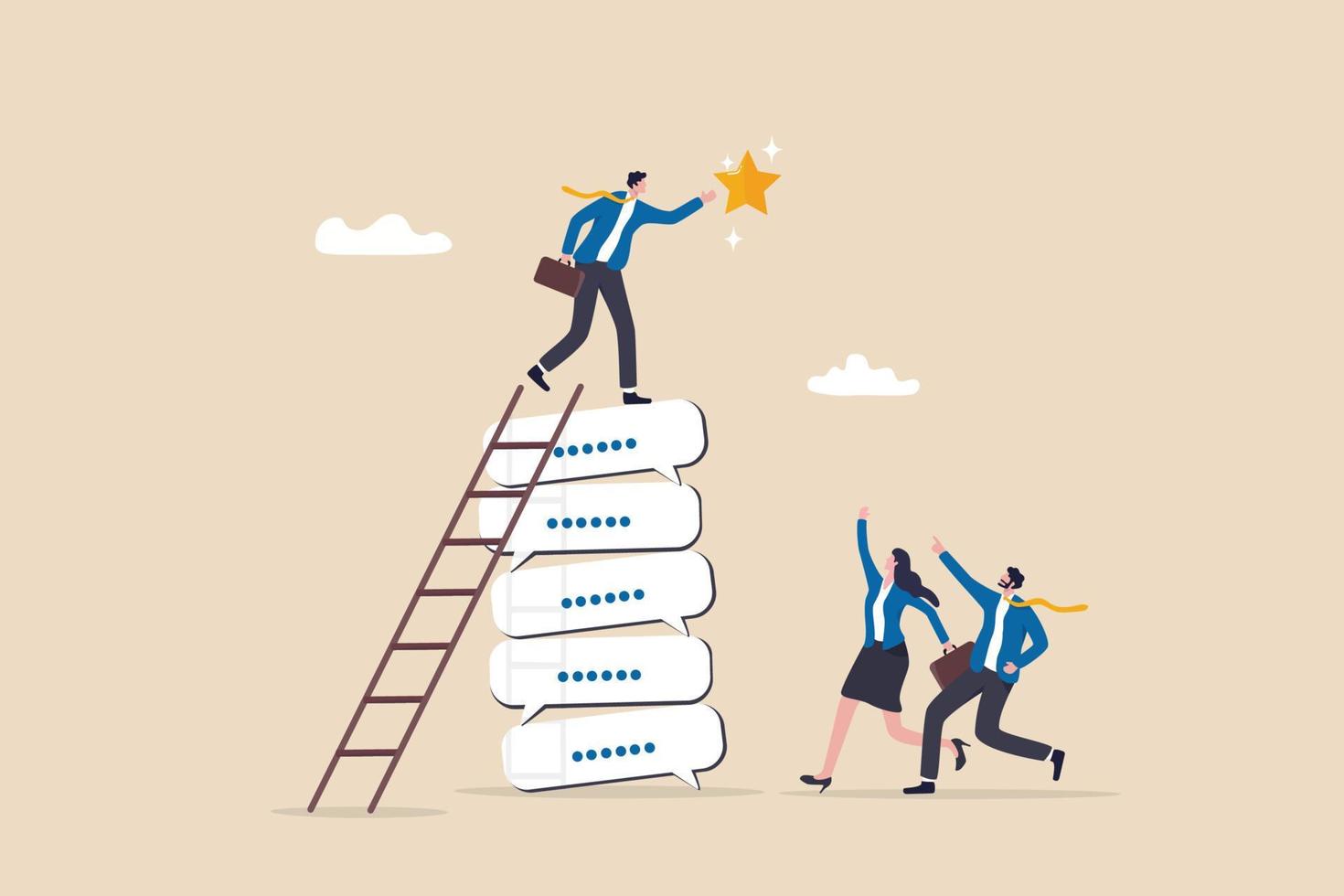This image, a minimalistic vector illustration, depicts a man reaching the top of a ladder made up of five text bubbles, each with typing dots, against a tan background with two scattered clouds and a star. The man, dressed in a blue blazer, white shirt, yellow tie, and black pants, is poised at the top, attempting to touch a golden star surrounded by white sparkles. He has black hair and his tie flows in the wind. At the bottom, two other individuals, one male and one female, similarly dressed in business casual blue blazers, white shirts, yellow ties, and dark pants, are waving and seemingly running towards the man, looking up and pointing at him.